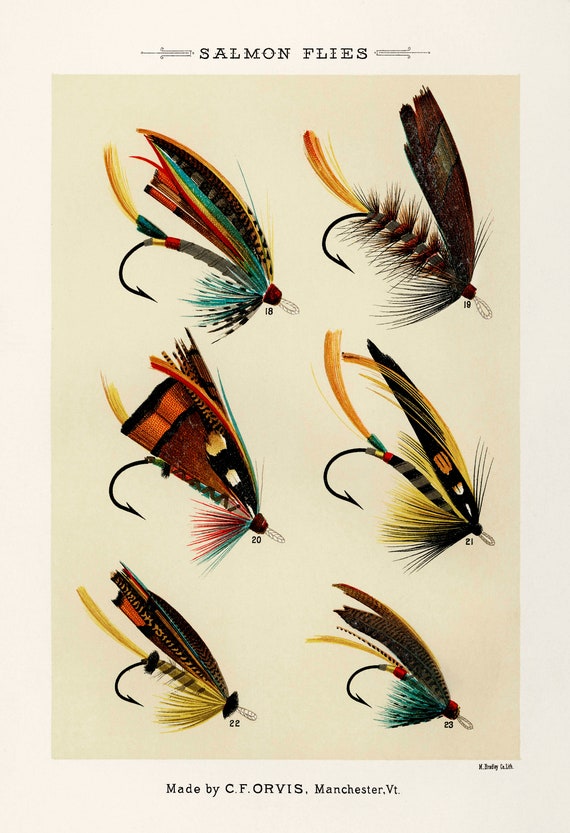The image titled "Salmon Flies" features six intricately crafted fishing lures made of feathers, neatly arranged in two columns and three rows. Each lure is unique in design and color, showcasing the artisan's skill. At the very top, in black text, the title "Salmon Flies" elegantly introduces the collection. Correspondingly, numbers 18 through 23 label the lures, from the top left to the bottom right.

The top left lure is adorned with green and black feathers and finishes with a black sharp hook. Adjacent to it is a lure featuring burgundy red feathers. In the middle row, the left lure resembles a butterfly, while its companion on the right is more predominantly yellow. The bottom row holds a yellow feathered lure on the left, and the rightmost lure mirrors the top left but adds variations: it has yellow and black feathers, a long brown feather, a green feather below, and a black hook on the left.

The lures are displayed on a yellow background, complementing their vibrant colors. The backdrop of the entire image features a peach or pink shade, providing a pleasing contrast and further elevating the presentation. At the bottom edge, black text reads, "Made by CFOVS Manchester VT," while some indiscernible text marks the bottom right corner.